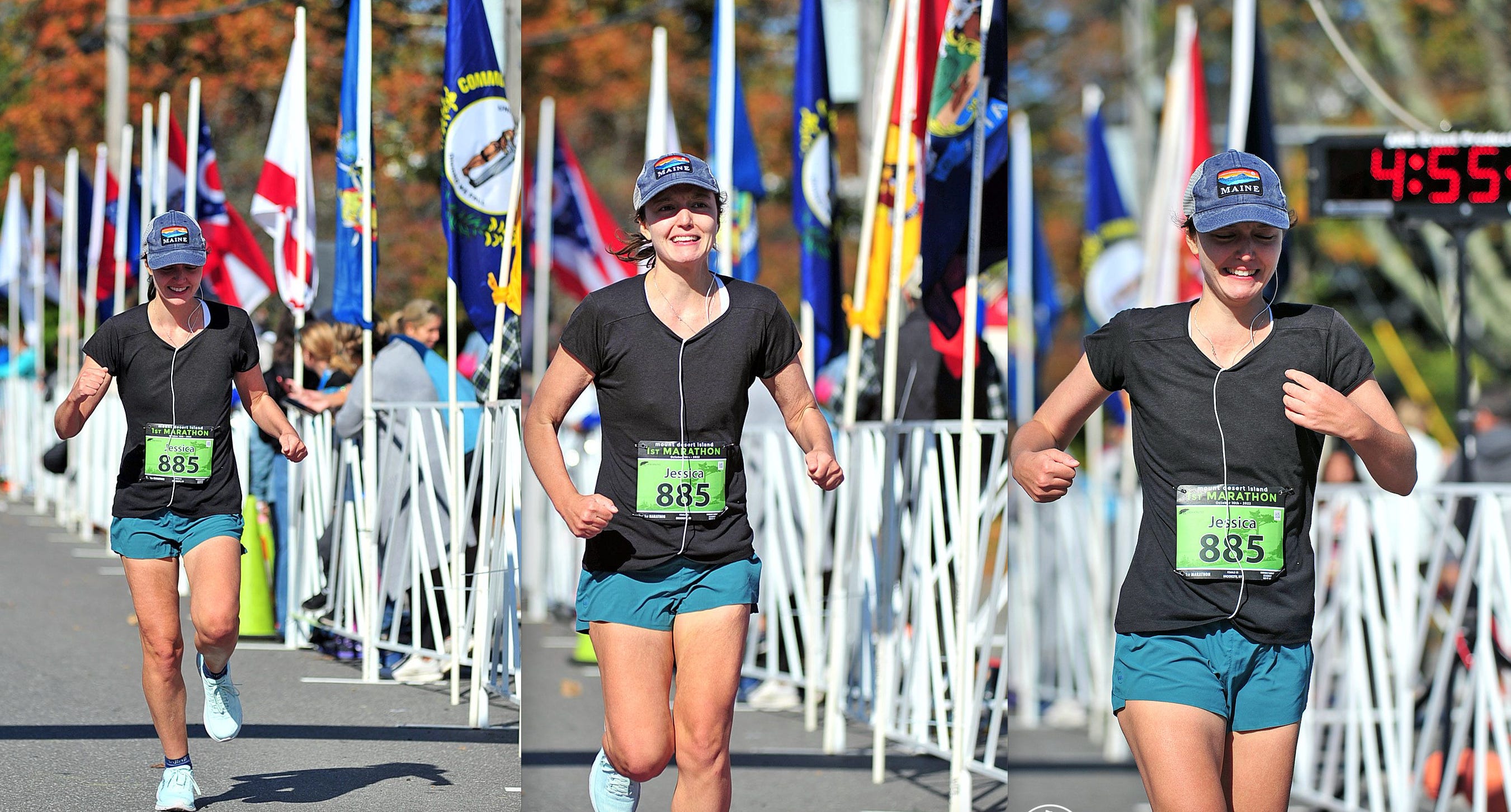The image shows a time-lapse sequence of a woman named Jessica running and progressively getting closer to the finish line of what appears to be a short, one-mile race. The race time visible on a clock in the images is 4.55, which may be her completion time. Jessica is wearing a race number 885 with a green badge, a black v-neck t-shirt, teal (or marine blue) jogging shorts, and white running shoes. She also has a white iPod cable visible under her t-shirt. Additionally, she sports a dark blue baseball cap with the word "Maine" on it. Behind her are autumn trees with vibrant red foliage, a white fence lining the race track, and an assortment of international flags. In each subsequent image, Jessica moves closer to the camera, transitioning from a focused to a smiling expression by the final shot, indicating her satisfaction or accomplishment in finishing the race. The presence of spectators and closed-off roads underscores the event's organized nature.